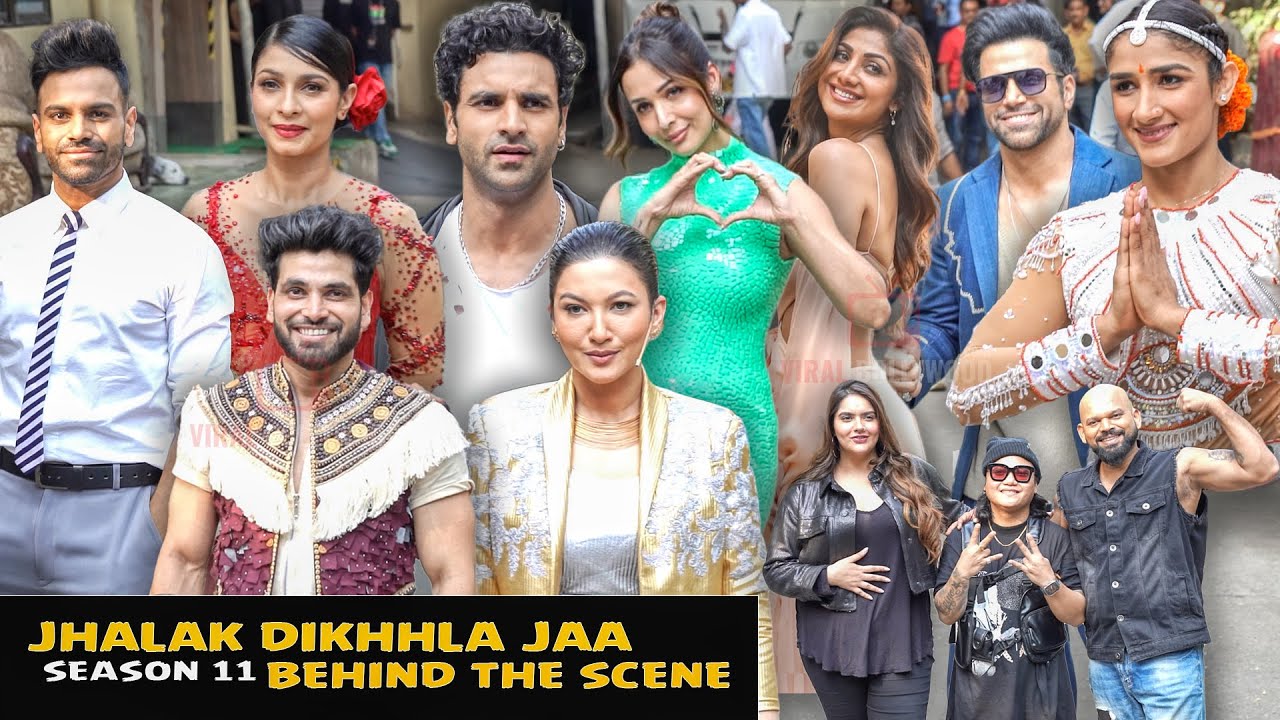The image is a promotional piece for an Indian television show, prominently featuring a collage of multiple individuals seemingly photoshopped together. The text within a black box at the bottom left corner reads "Jhalak Dikhhla Jaa, Season 11, Behind the Scene," with "Jhalak Dikhhla Jaa" and "behind the scene" in gold color while "Season 11" is in white. The image showcases a multitude of people, many of whom are dressed in elaborate Indian attires and diverse outfits reflecting both traditional and contemporary styles.

On the left side of the image is a man dressed in a white shirt with a striped tie, paired with gray pants, standing next to a woman in a red dress adorned with a red flower in her hair. Nearby, there is a man with poofy brown hair and a beard, wearing a distinct purple garment with white fringe. Another woman, seen in a green dress, is making a heart shape with her hands.

In the bottom right of the image, three individuals who seem to be unrelated or possibly judges are dressed in black. One is a bald man in blue jeans and a black shirt. Another is a young man making a peace sign, and the third is a woman with long brown hair, her hand placed over her stomach. They all are smiling and looking directly at the camera. The image captures a vibrant array of personalities and styles, likely from different scenes or promotional shots of the show.